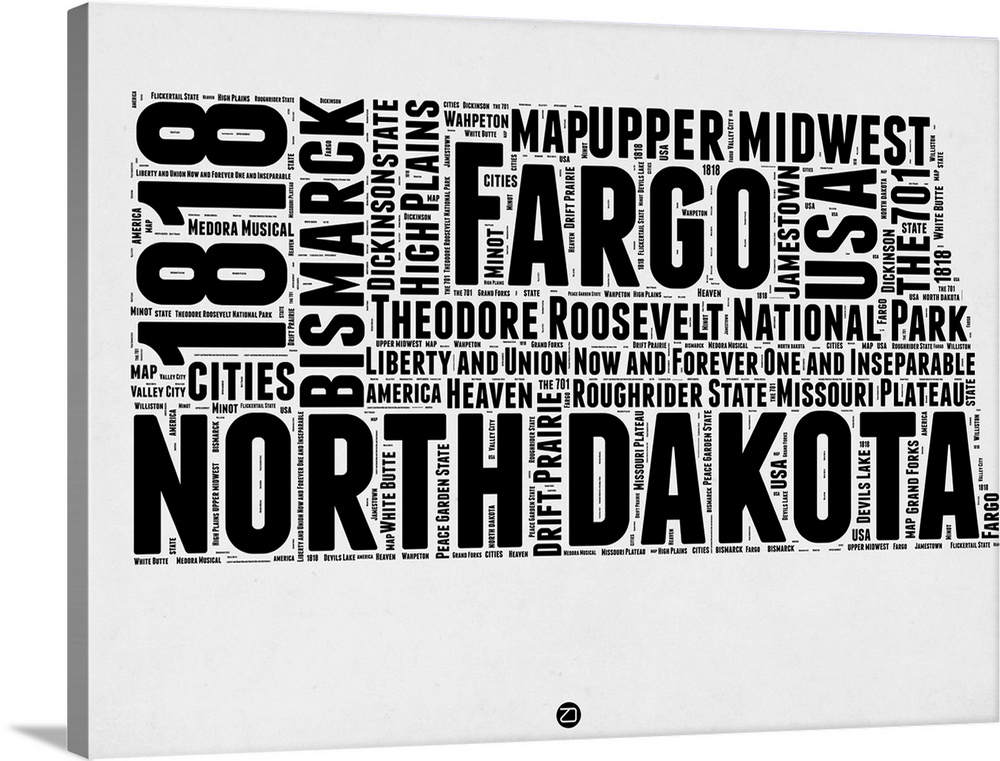The canvas art piece has a white background adorned with a black font showcasing the names of different cities and regions, predominantly focusing on North Dakota and its attributes. Across the canvas, words are arranged both vertically and horizontally, with larger and bolder capitalized names such as "North Dakota," "Fargo," "1818," "Upper Midwest," "USA," and "Theodore Roosevelt National Park" standing out prominently. These significant terms are central and easy to spot, emphasizing key elements associated with North Dakota. The canvas also features smaller and less spaced words, including "Bismarck," "Liberty and Union, Now and Forever, One and Inseparable," "America," "Heaven," "Roughrider State," "Missouri Plateau," "Drift Prairie," and "Peace Garden State." The densely packed fonts vary in size, with some words being so small they are hard to read, creating a textured and dynamic word cloud effect. At the bottom, a small black circle with an unidentified white logo adds a subtle finishing touch to the composition, affirming the piece's intricate visual tapestry of North Dakota's identity.